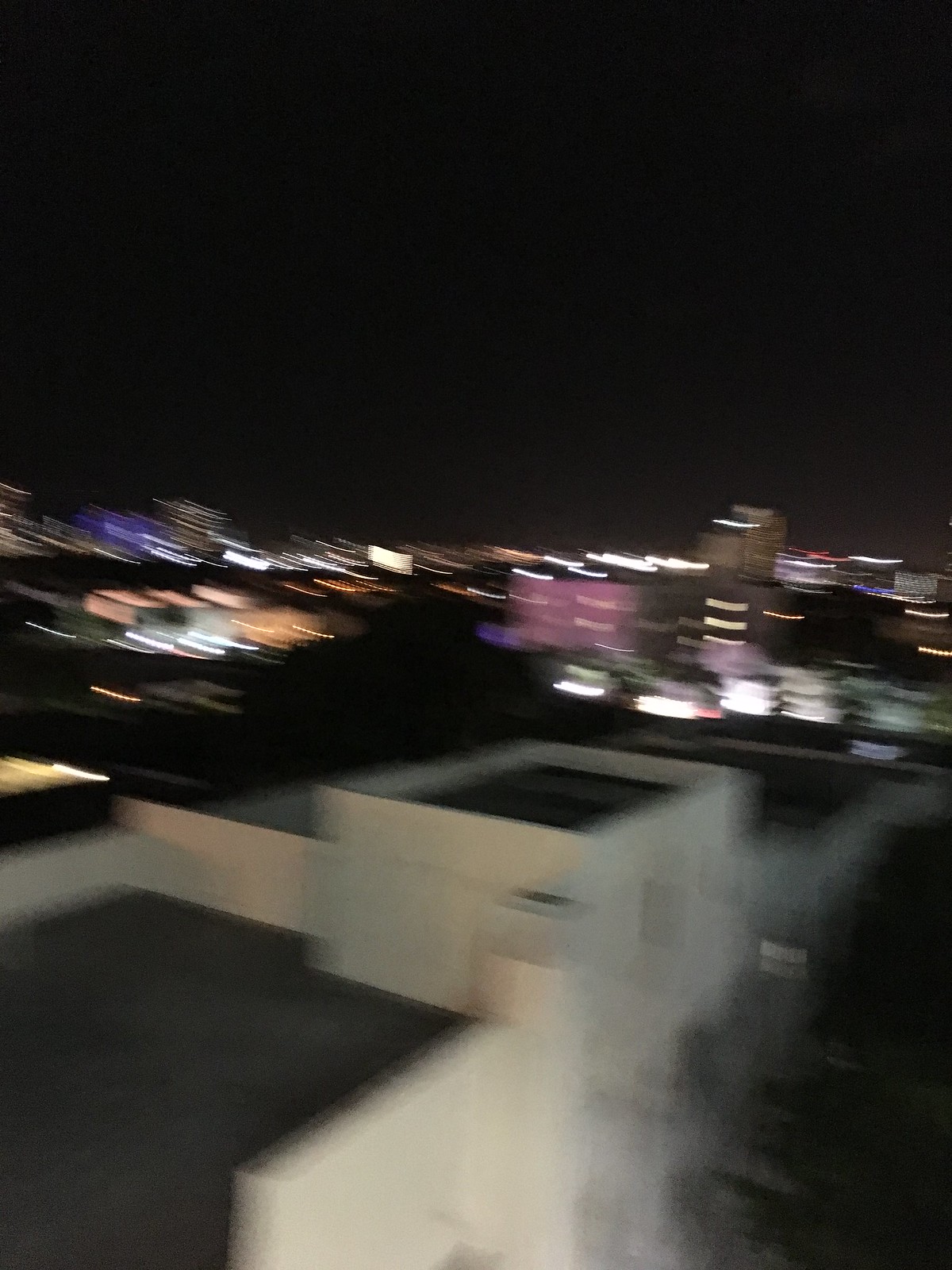This is a very blurry night photograph taken from the rooftop of a white building with black floors in the middle of a city. The dark sky occupies the top of the image, while the foreground features part of the white building with its black rooftops. The cityscape stretches out below, filled with a tapestry of blurred, colorful lights—shades of pink, white, green, purple, orange, and yellow. These lights, emanating from various urban structures like shopping centers, apartment buildings, and office buildings, seem to shift horizontally across the picture, obscuring specific details and creating a diffuse, dreamlike effect.